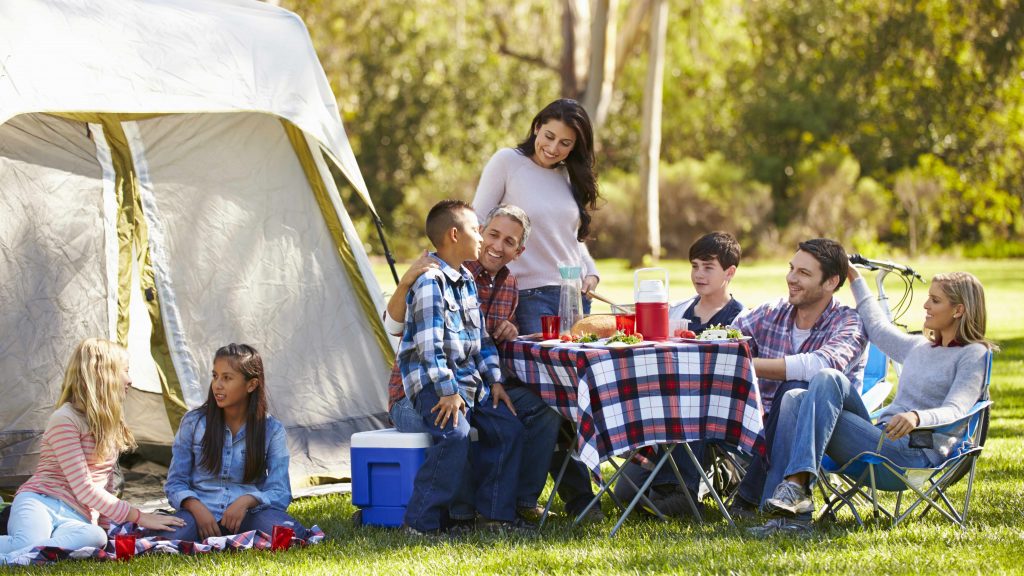This vibrant color photograph captures a lively family camping scene on a sunny day. Situated in the great outdoors, the image shows eight people reveling in each other's company. To the far left, a white tent with a partially open flap serves as a backdrop for two girls seated on the ground in front of it. One girl, with blonde hair, is dressed in a red and white striped shirt and white pants, while the girl beside her has long dark hair draped over her shoulders, donning a blue long-sleeved shirt and jeans.

The central focus of the image is a portable table adorned with a checkered tablecloth and laden with an array of food items, red Solo cups, a small thermos, and pitchers of beverages. Six people surround the table, two of whom are perched on a blue cooler. On one side, a man and a young boy—both smiling—enjoy the moment. The man is in his late 20s, laughing heartily, while the boy looks forward intently.

On the opposite side of the table, a young boy sits next to a woman who exudes joy, standing and smiling warmly at the people seated. She wears a white or cream sweater, blue jeans, and her presence further enlivens the atmosphere. Adjacent to her, a woman in flannel clothing, seated comfortably in an outdoor lounge chair, shares a touching moment with a man seated next to her, her right hand resting gently on the back of his head. 

A bicycle can be seen to the right of the scene, adding to the authenticity of the camping environment. The photograph captures a snapshot of pure happiness and familial bond, with every individual engaged in cheerful conversation and laughter.